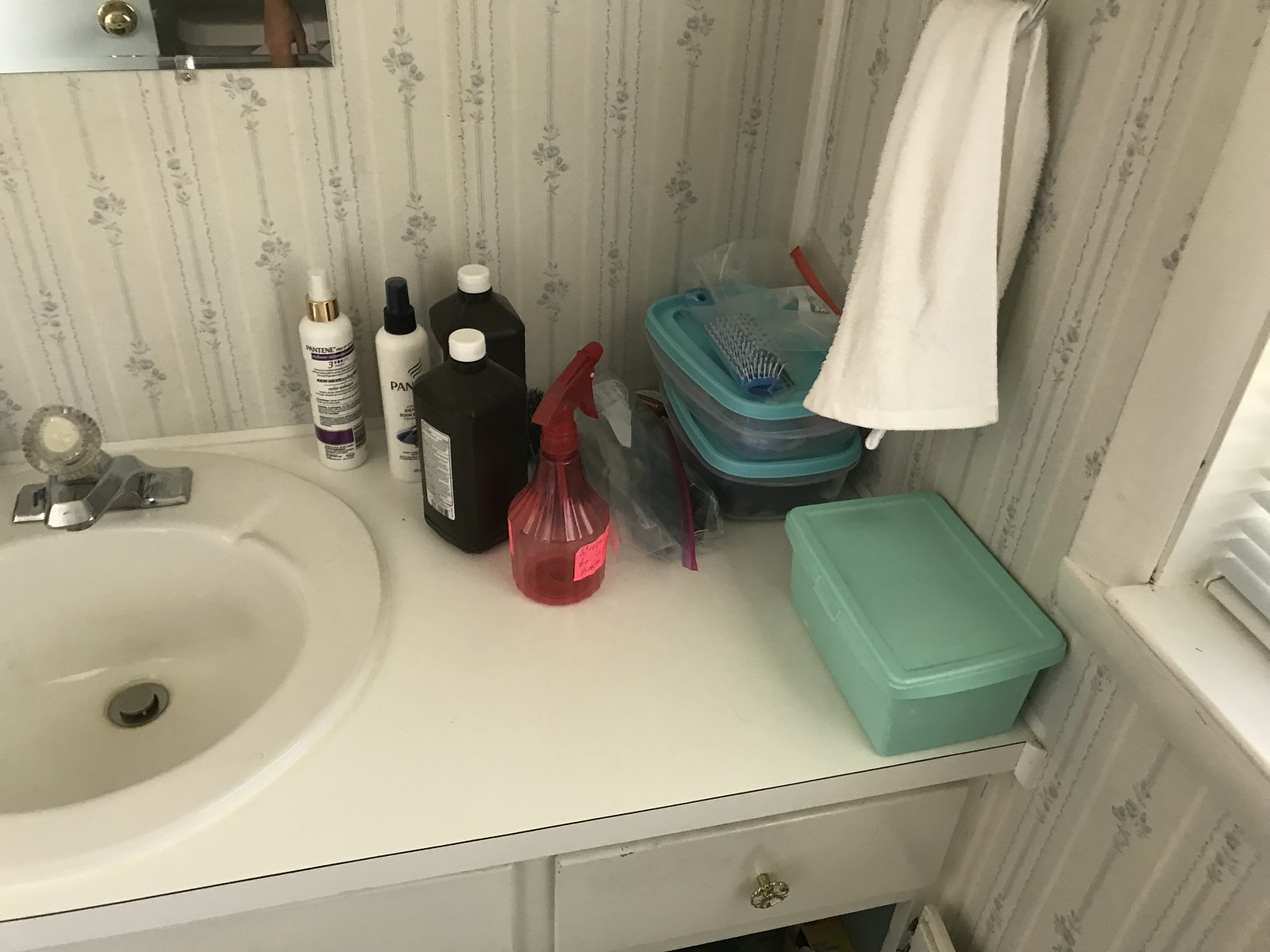This photograph depicts a vintage bathroom, with evident signs of its age in various elements throughout the space. The windowsill exhibits noticeable wear and tear, adorned with dated Venetian blinds on the right side. The sink area features a white, sharp-edged material distinctive of older designs, alongside a 1980s-style surface-mounted rim sink and corresponding faucet. The mirror on the wall is supported by clips that hint at styles from the 1970s or 1980s. The wallpaper, however, appears more contemporary, contrasting with the overall retro aesthetic.

The cabinetry below the sink, including drawers and a bath unit, is marked by worn drawer knobs and visible bumps and bruises, characteristic of designs from several decades ago. In terms of decor and utilities, various items are scattered atop the counter: a bottle of Pantene shampoo, a bottle likely containing alcohol or an antiseptic solution, a green tote, a hairbrush, and a couple of other plastic containers. These details collectively contribute to the nostalgic atmosphere of this quaint bathroom.